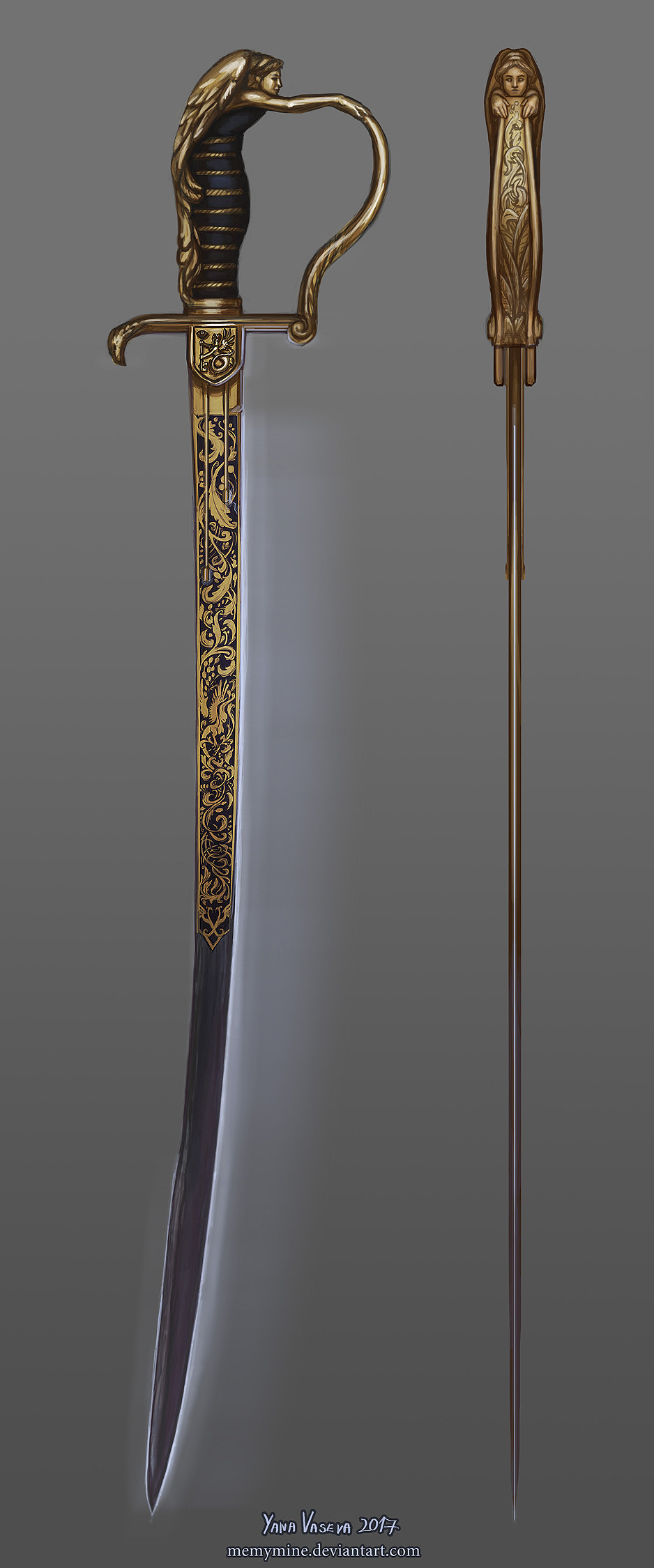This photograph captures an intricately designed sword, shown from two different angles against a dark grey background in a vertical rectangular frame. On the left, the side view reveals a long, thin blade made of dark grey steel with ornate, gold and black engravings that resemble leaves and feathers on the top half. The blade tapers to a point and has a slight curve. The handle, positioned at the top, features a bronze or dark brass depiction of a woman with long hair extending into the curved handguard, her arm outstretched to form the curve. The hilt includes detailed facial features and transitions into a flat base before the blade starts.

On the right side of the image, the top view further details the ornate handle design where the woman's sculptural form continues, her wings and hands cradling the base in an elegant, scrolling motif done in black and gold. This detailed craftsmanship extends along the blade with additional engravings. The image includes text at the bottom, indicating "Uneva Manson 2017" and a DeviantArt website, highlighting the modern creation of this antique-looking piece.